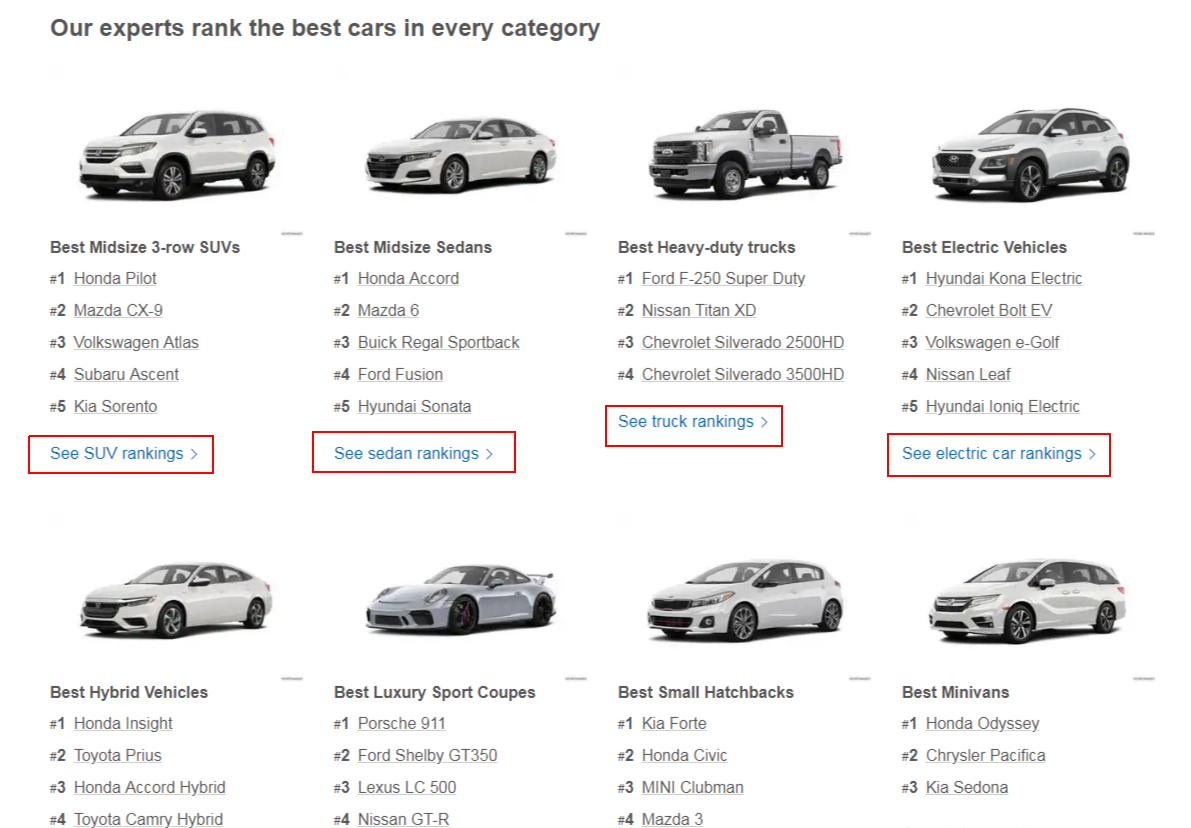The image depicts an automobile website with a pristine white background. At the very top, there is a clear, bold black text that states, "Our experts rank the best cars in every category." Below this title, the page is divided into two rows of vehicles, each consisting of four vehicles, totaling eight across the entire page.

In the top row, each vehicle is showcased in a white or gray color scheme. The first vehicle is a white Honda Pilot, designated as the "Best Midsize Three-Row SUV." Next to it is the "Best Midsize Sedan," followed by the "Best Heavy-Duty Trucks," and finally the "Best Electric Vehicles." Each vehicle category includes a link beneath it, outlined in a red-colored box, inviting viewers to "See SUV rankings" or respective rankings.

The bottom row continues with the "Best Hybrid Vehicles," followed by the "Best Luxury Sport Coupes," the "Best Small Hatchbacks," and concluding with the "Best Minivans."